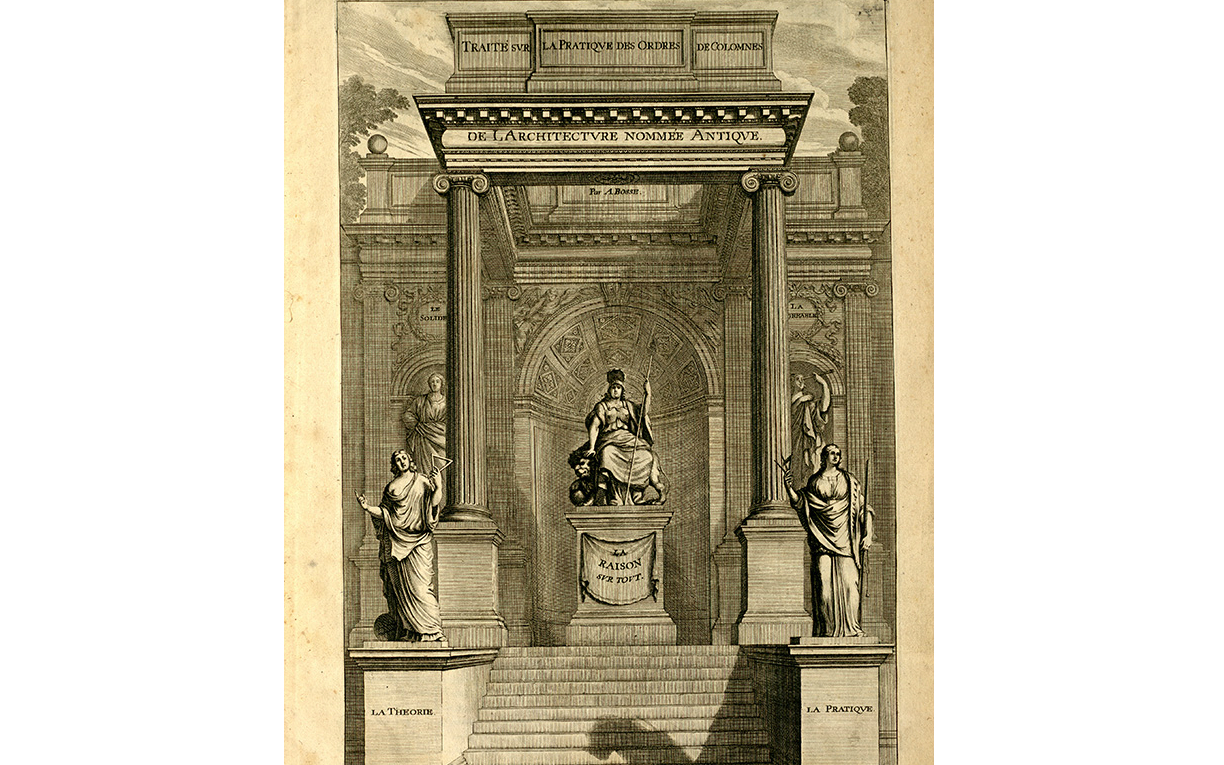The image is an intricate black and white engraving, likely inspired by ancient Greek or Roman designs, depicted on light brown paper or papyrus. It features a central statue of a seated figure on a throne, draped in robes, holding a scepter, and wearing headgear that might be a helmet adorned with a feather plume. This main statue is situated on a pedestal, looking outwards from the structure. Surrounding the central figure is a grand architectural setup with multiple pillars and descending steps in front. 

Flanking the staircase are two prominent statues of men, each holding mathematical symbols, with one additionally wielding a lance. Behind these figures are further pillars, each topped with statues of robed individuals. French inscriptions are visible across the artwork: "Architecture Gnome Antique" prominently above the central pillars and statues, "raison surto" suggesting "reason over everything," and smaller texts like "la théorie," "la pratique," "la solidarité," and others that are partially illegible.

The overall scene appears to be an elaborate and symbolic portrayal, celebrating both architectural grandeur and intellectual virtues through its detailed and meticulously arranged elements.